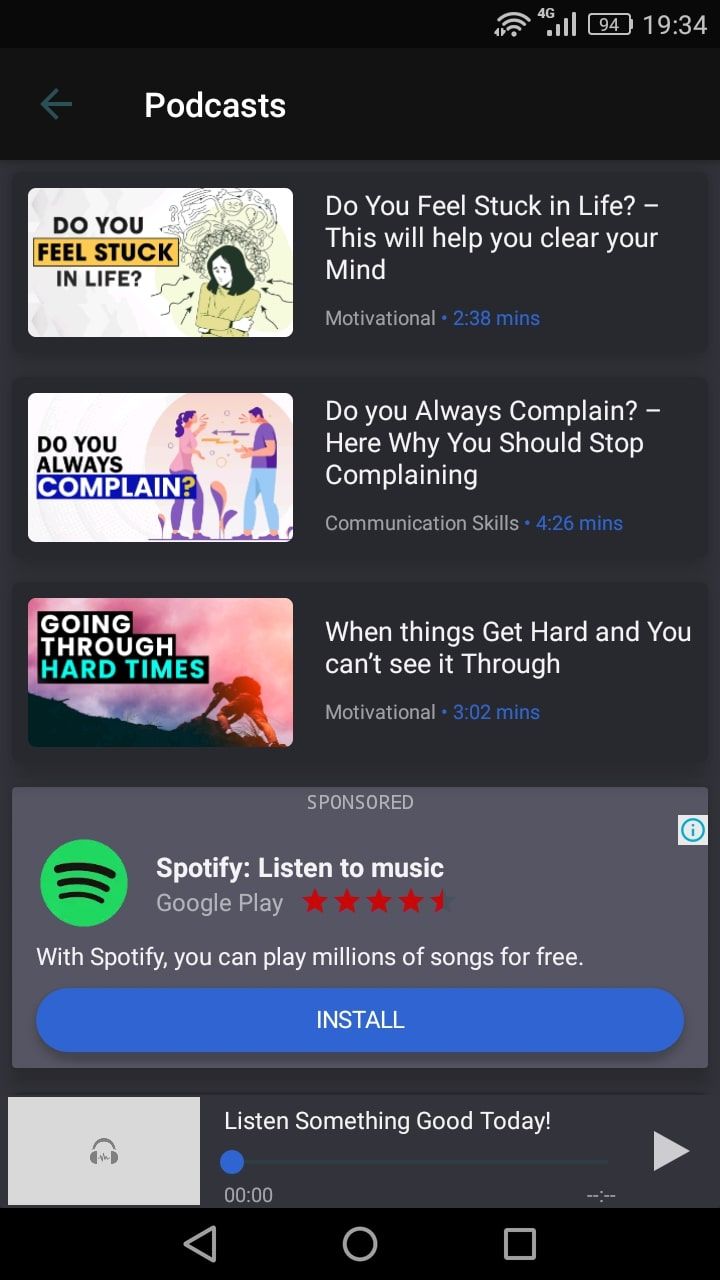This detailed caption accurately describes the content of the screenshot:

The image is a screenshot from a mobile device, depicting a podcast application interface. At the top of the screen, various status icons are visible, indicating Wi-Fi connection, network connection, battery status, and the current time. The main section of the app is labeled "Podcasts" and includes a back arrow for navigation to previous pages or the home screen.

The screenshot displays a list of three podcasts. Each podcast entry features a thumbnail image on the left side, accompanied by a title, a category, and a duration. For example, the first podcast is titled "Do you feel stuck in life? This will help you clear your mind", categorized under "Motivational", and has a length of 2 minutes and 38 seconds.

Below the list of podcasts is a sponsored advertisement for Spotify, providing an option to install the app. Additionally, the current podcast or music track playing is titled "Listen Something Good Today."